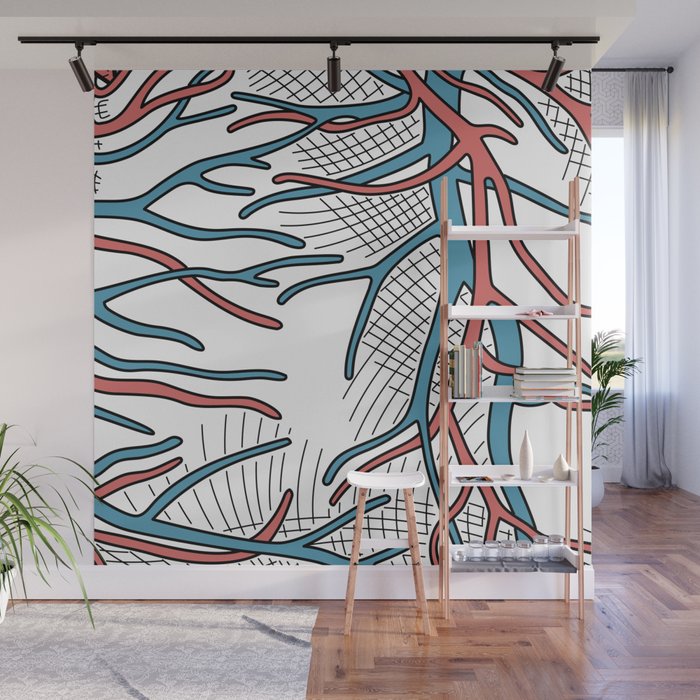The photo captures a chic and modern living space inside a house or apartment. The room's focal point is an intricate wall design that features an abstract mural resembling veins or roots, in blue and reddish-pink hues with black outlines, set against a clean white background. This mural spans from the ceiling to the baseboard, creating a striking artistic effect enhanced by the track lighting above. A tall, narrow bookshelf with a wooden frame and white shelves stands to the right of the wall, while a matching stool with thin wooden legs and a white seat is positioned to its left. The floor is wooden, adorned with a simple gray rug, and the baseboards are white. In the distance, a partial view of another room reveals white curtains, a window, and a houseplant in a white pot. The entire space exudes a minimalist and stylish atmosphere.